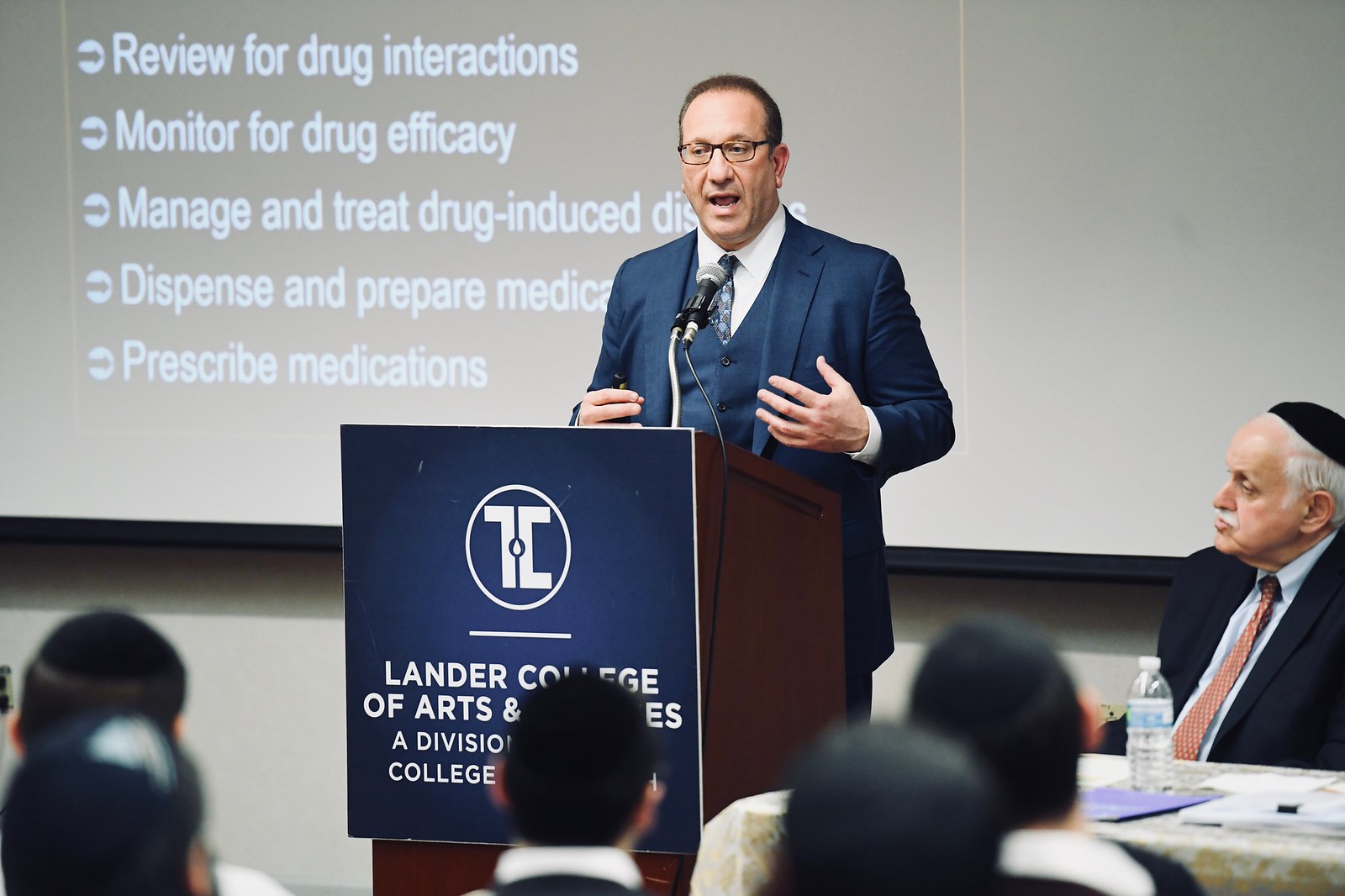The image features a man standing at a wooden lectern, giving a lecture and speaking into a microphone. He is dressed in a blue three-piece suit, a white button-up shirt, a blue and green tie, and glasses. His left hand is raised in a gesture as he speaks. Behind him, a PowerPoint slide projected on a screen displays partial text, including "Review for Drug Interactions," "Monitor for Drug Efficacy," "Manage and Treat Drug-Induced," "Dispense and Prepare Medications," and "Prescribe Medications." The slide's text is partially obscured by the man at the lectern. The lectern itself has a sign that reads "Lander College of Arts and Sciences, a division college," though some words are blocked by the people sitting in the front row. To the left of the speaker, another man is sitting near a table, wearing a yarmulke and a blue suit with a red tie, with a bottle of water in front of him.